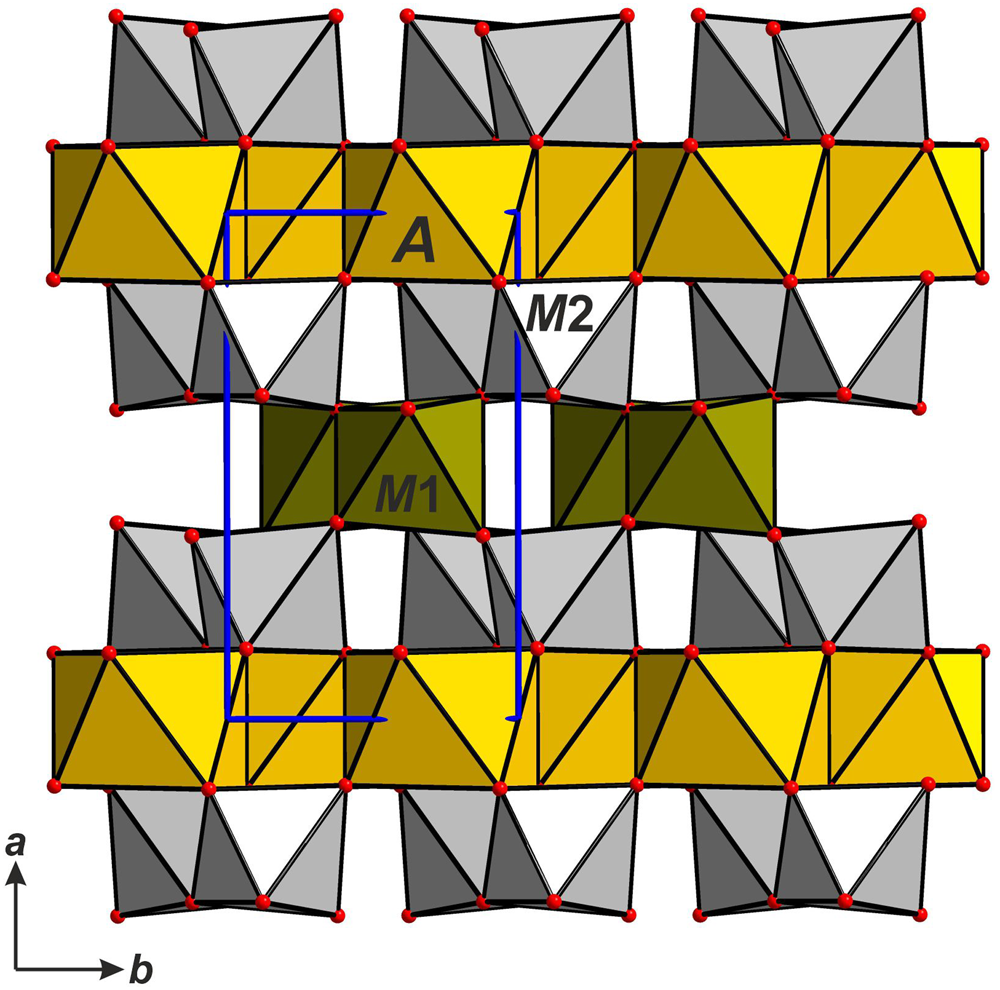The image is a detailed drawing featuring an intricate assembly of geometrical shapes connected in a seemingly complex structure. Primarily composed of triangles, these shapes are formed with black lines and filled with different colors including gray, yellow, green, and white. Within each of these shapes, additional black lines intersect, terminating in red dots. Several geometric figures include labels such as A, M1, and M2, adding to the diagram's complexity. 

The overall structure appears as a series of interconnected triangles, creating a 3D effect reminiscent of cubes stacked together. Of particular note, one triangle labeled A appears in the upper golden section, M2 in the center of the silver section on the third row, and M1 in the second square of the olive-colored middle row. 

At the bottom left corner of the drawing, two black arrows are positioned perpendicularly, denoting axes labeled A (vertical) and B (horizontal). The entirety of this intricate design is set against a white background.